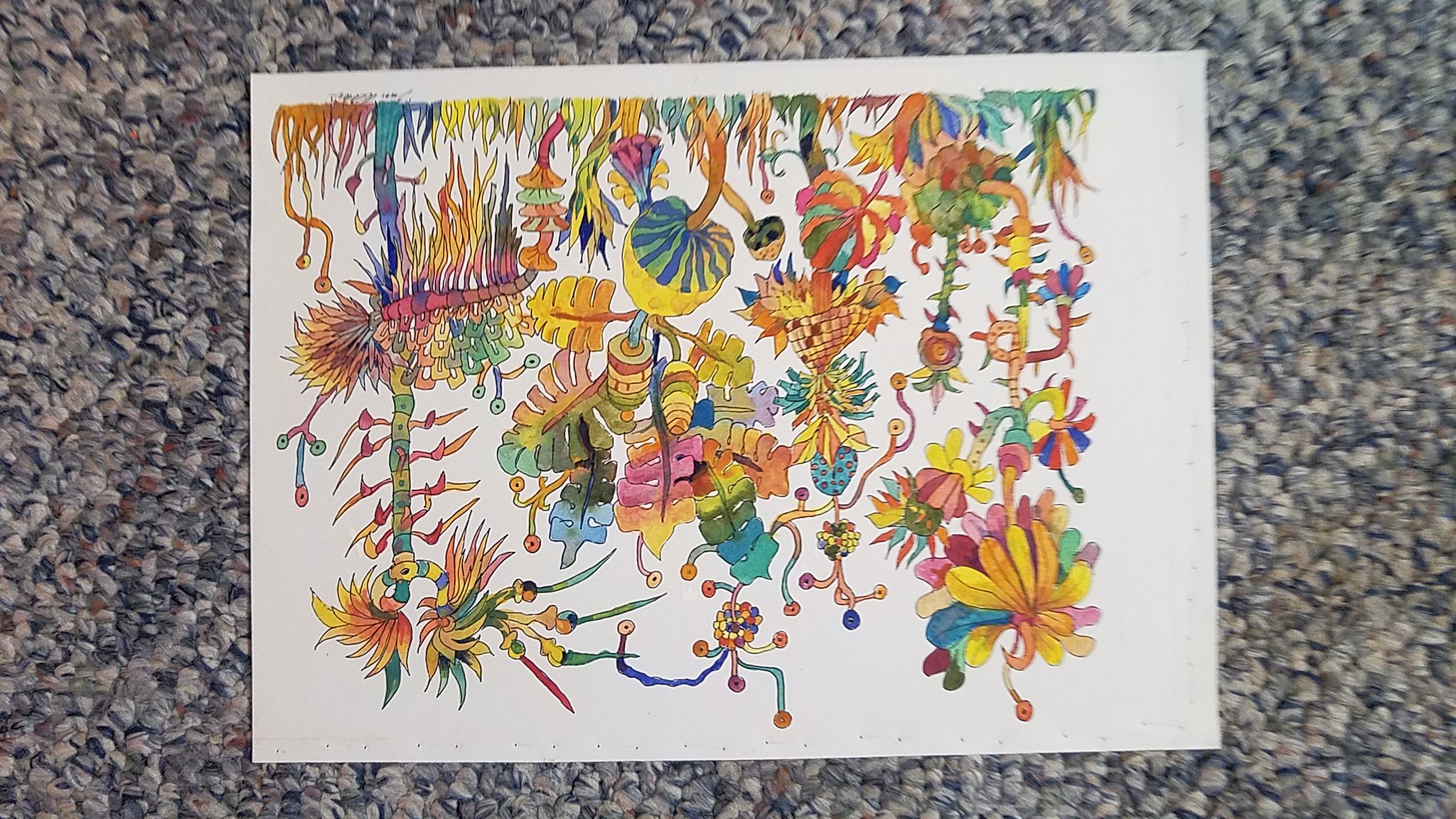This color photograph captures an intricately detailed drawing, currently placed upside down, on a textured, tweed-like grayish carpet that features mingled tones of beige, gray, and off-white. The drawing, rendered on white paper in an oblong shape, appears vibrant and cheerful with a multitude of colorful plants, mushrooms, and trees depicted in a whimsical and fanciful style. Despite its inverted position, the composition remains visually engaging and pleasing, showcasing the artist's attention to detail and creative execution.